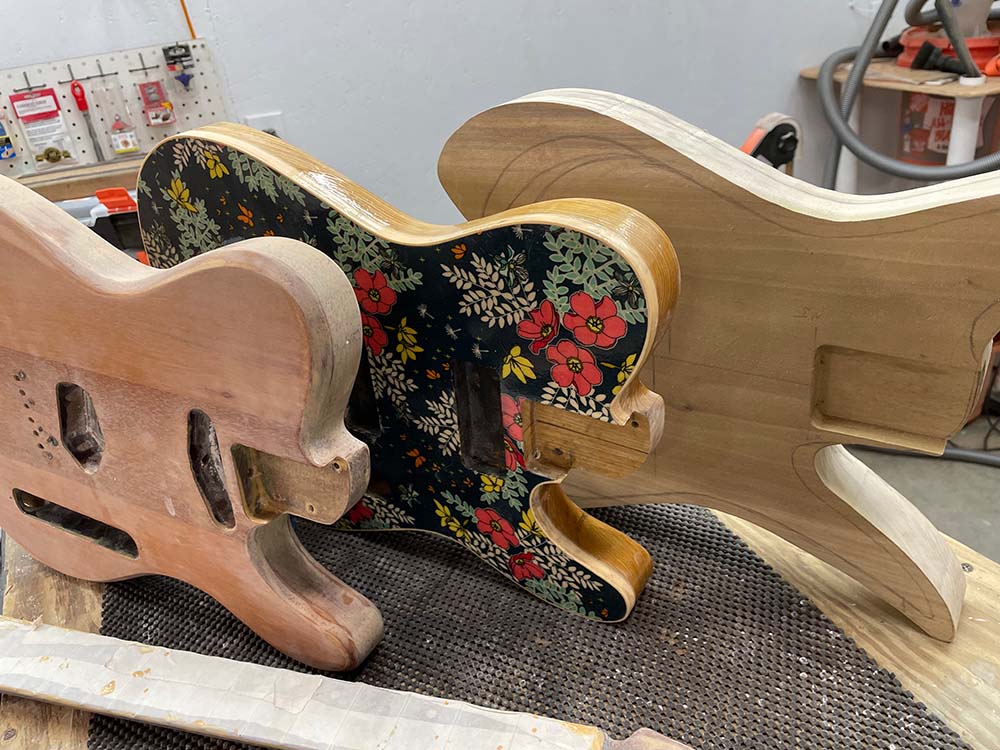This image depicts three half-finished wooden electric guitar bodies standing on their sides on a wooden surface with a black non-skid pad. Behind them is a white wall adorned with a pegboard filled with tools, and a shop vac is visible, indicating a workshop setting. From left to right, the first guitar body is made of reddish wood and features cut-out holes for the handle and fretboard; it appears unfinished as it lacks stain or any finishing details. The central guitar body stands out with its decorative floral print comprising pink, yellow, blue, red, and beige flowers against a black background. The guitar body on the far right is the most raw, with visible pencil markings on its fresh, unstained wood. The overall scene conveys an artisan workspace mid-project.